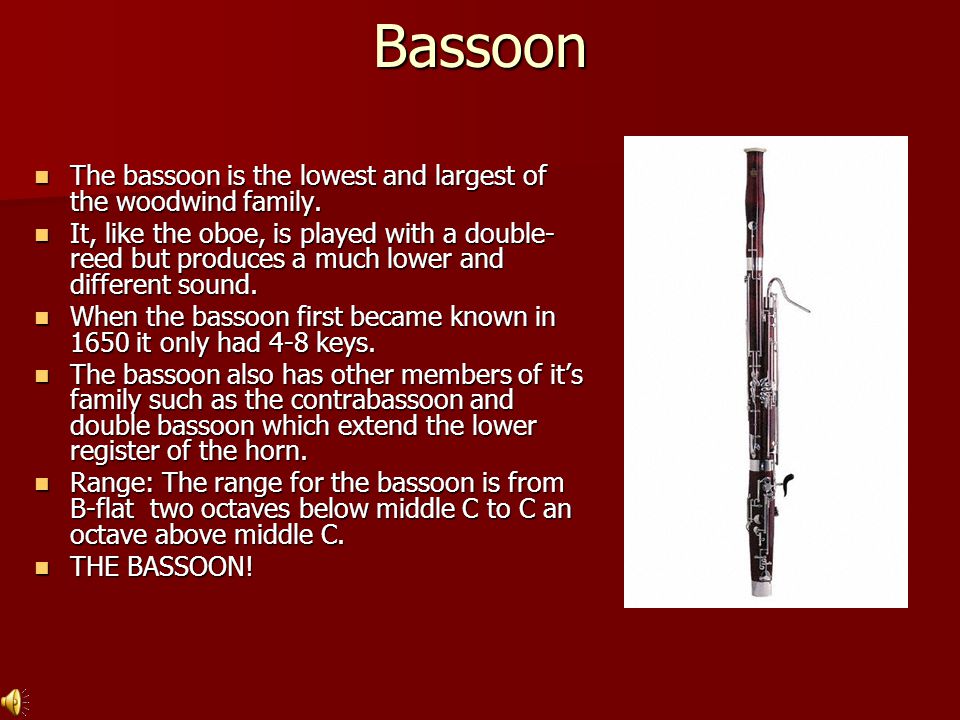This image is a horizontal rectangular PowerPoint slide focused on the bassoon, a woodwind instrument. The slide has a deep maroon background with a white section occupying the right third of the slide. In the white section is an image of a black bassoon with silver piping, including a silver reed protruding from it. The title at the top of the slide reads "Bassoon" in large, whitish-yellow text. The left two-thirds of the slide features a bulleted list in white text that describes the bassoon’s attributes. The bullet points highlight that the bassoon is the lowest and largest member of the woodwind family, played with a double reed like an oboe but producing a much lower and distinctive sound. It mentions the bassoon's origins in 1650 when it had only four to eight keys, and notes the existence of other bassoon family members such as the contrabassoon and double bassoon, which extend the instrument’s lower range. It specifies the bassoon's pitch range from Bb, two octaves below middle C, to C, an octave above middle C. The final bullet point emphatically states 'THE BASSON!' in all caps. A small speaker icon is located in the lower left corner, suggesting that clicking it would likely play a sample of bassoon music.